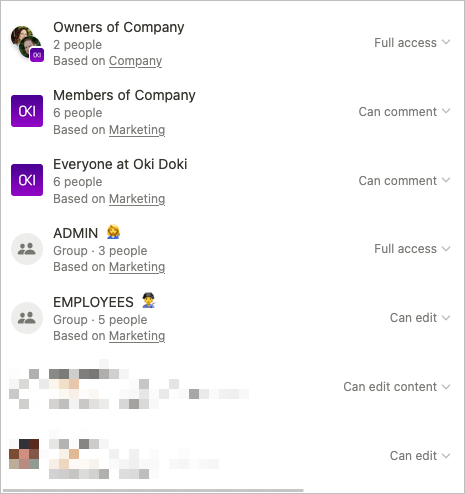Screenshot of Permissions Menu for Okidoki Company Website:

The screenshot displays a permissions menu for a company, presumably Okidoki. The menu features a clean, white background with primarily black or gray text unless otherwise specified. 

- **Owners of the Company:** Two individuals, designated under the category 'company' (underlined), have full access to all features.
- **Members of the Company:** Six individuals under the 'marketing' category can comment on content.
- **Everyone at Okidoki:** Similarly, six individuals under the 'marketing' category are granted commenting permissions.
- **Administration Group:** This group comprises three people from 'marketing', who possess full access privileges.
- **Employees Group:** Five individuals from the 'marketing' team have the ability to edit content.

The last two groups are blurred out and heavily pixelated, but their permissions are noted as 'can edit content' and 'can edit,' respectively.

This detailed permissions menu is likely part of the settings for a company's forum or website, indicating different access levels across various user categories.